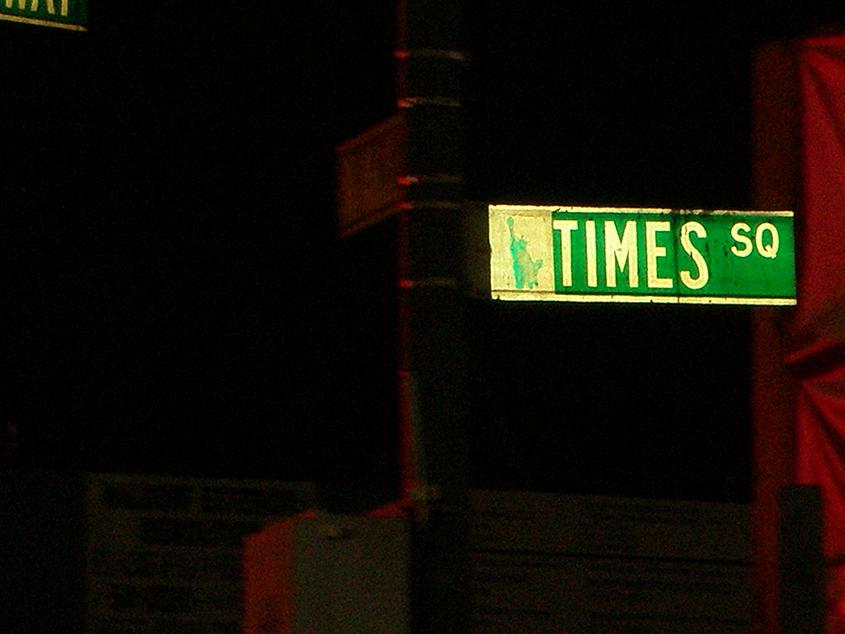This nighttime photograph captures a dimly lit urban scene dominated by shadows, with only a few elements illuminated. On the right side of the landscape-oriented image, an illuminated green street sign stands out prominently. The sign, which indicates "Times SQ" in yellowish-white letters, glows brightly against the dark backdrop, suggesting it's a directional sign for Times Square, New York City. The left part of the sign features a white square with a stylized image of the Statue of Liberty, characterized by a greenish outline and a whitish front, with the torch extending upwards.

Attached to this sign is a vertical, black pole with slight silver reflections from horizontal straps securing the sign. There is also a hint of another street sign pole nearby, and indications of a few red squares, possibly reflections or objects, peeking from the right side of the frame. A partially visible box, likely a pedestrian crossing button, is affixed to the pole but mostly obscured by shadows. Behind this setup, parts of a brick building can be faintly discerned in the poorly lit background, adding to the urban ambiance of the scene.